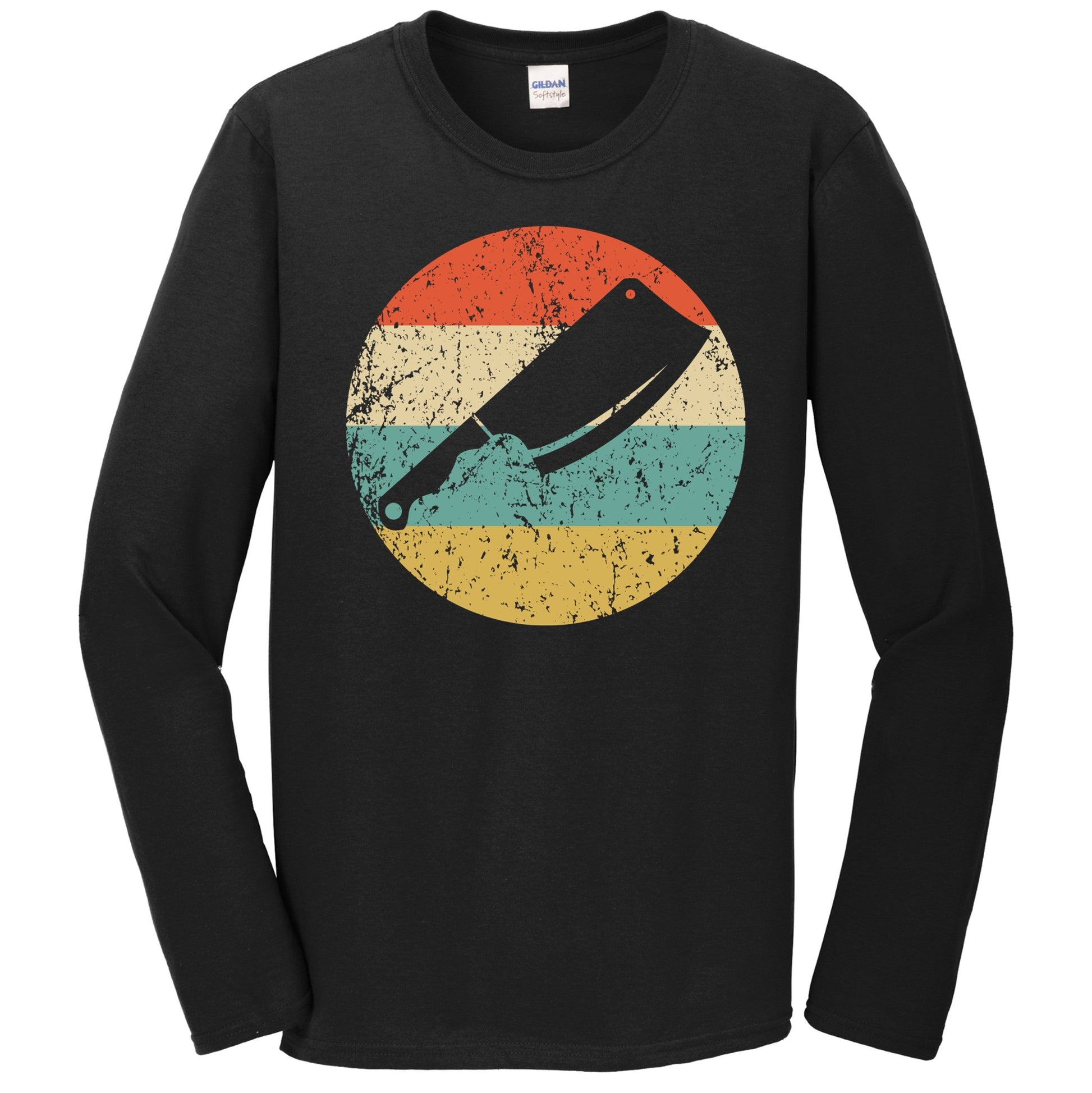The image depicts a black long-sleeved sweatshirt made from cotton material, laid out on a white background. The sweatshirt features a round neck and has long sleeves that are bent inwards. It bears a white tag inside with the brand "Gildan." Dominating the front of the sweatshirt is a retro-styled circular logo, positioned centrally on the chest. This logo is divided into four horizontal stripes of color: red-orange at the top, followed by cream, turquoise blue, and finally tannish-yellow at the bottom. Superimposed over this colorful background is the outlined image of a black cleaver with a handle featuring circular cutouts both at the top of the blade and the end of the handle, giving it a vintage or rustic look with slightly faded, mottled details.